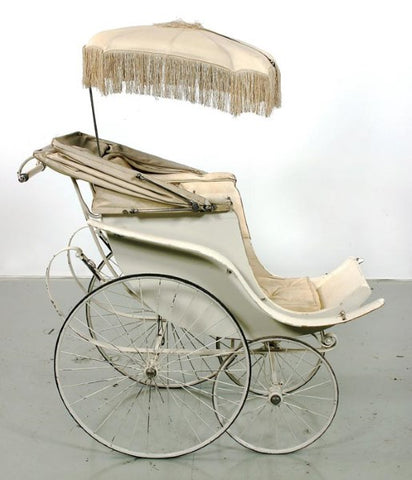The photograph depicts a nostalgic, old-fashioned baby carriage or pram set against a predominantly white background occupying the upper two-thirds of the image, transitioning to a grey or silver base. The carriage, reminiscent of a bygone era's horse-drawn buggies, prominently features four black wheels—the rear ones significantly larger than the front ones, with striking silver or grey spokes. This elegant white carriage boasts a cushioned seat with a luxurious tan or beige interior, enveloped in a touch of refined sophistication. Above, a lavish sun umbrella with delicate tassels adds an extra layer of grandeur, casting gentle shade over the seat. The overall aesthetic conveys a sense of vintage opulence and meticulous craftsmanship, indicative of something that would be manually pushed from behind.